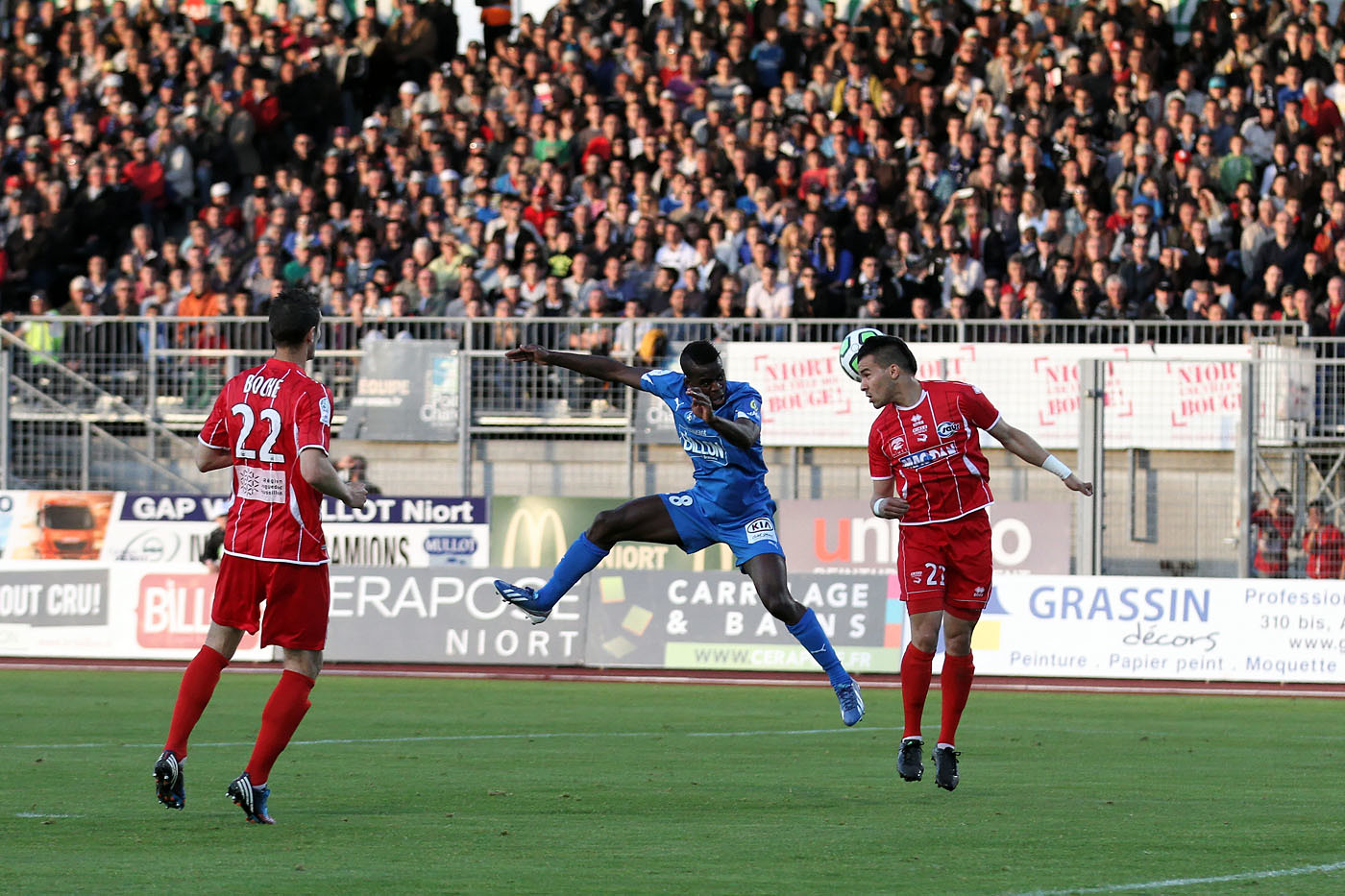The image captures an intense moment in a soccer match with three players in mid-action on a vibrant green grass field. Two players are dressed in red uniforms, complete with red jerseys, shorts, and socks. The player on the left, wearing the number 22, is leaping with only his right toe touching the ground, facing the player in blue at the center. The player in blue, dressed in a full blue kit, is airborne with his right leg high above. To the right, a red-uniformed player, number 23, with white stripes on his shirt, is about to make contact with the soccer ball using his head. Behind them, the stadium is bustling with thousands of spectators seated under the bright sun. A fence separates the stands from the field, and various advertisements adorn the wall beneath the crowd, including a notable yellow McDonald's "M" and another for Grasson Decors.